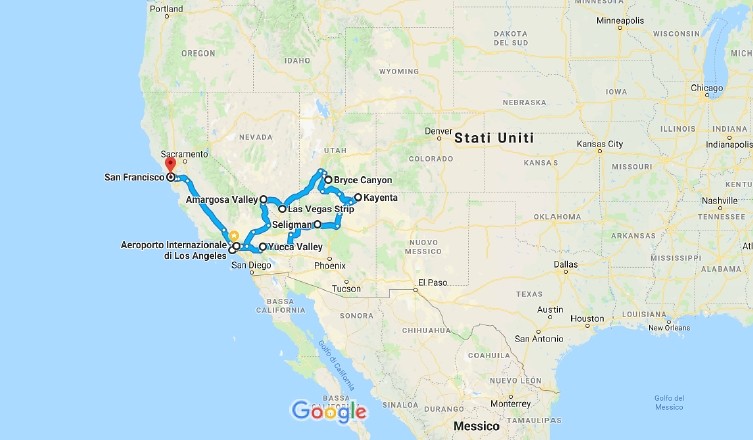This image depicts a detailed map highlighting specific regions in the United States and parts of Mexico. The map extends from Indiana, Kentucky, and Tennessee in the east, spans across Alabama, and reaches all the way to California, dipping just south of Monterey. It also includes portions of Mexico. The map background is predominantly white with light green accents, while state and city names are labeled in black. Centrally, the words "STATI UNITI" are inscribed. Surrounding the map, you can see water bodies, with notable paths drawn on it.

A prominent red marker indicates a route beginning in San Francisco, descending southward towards an airport in Los Angeles. The path intricately weaves around notable locations including Bryce Canyon, Kayenta, the Las Vegas Strip, Selma, and Yucca Valley.